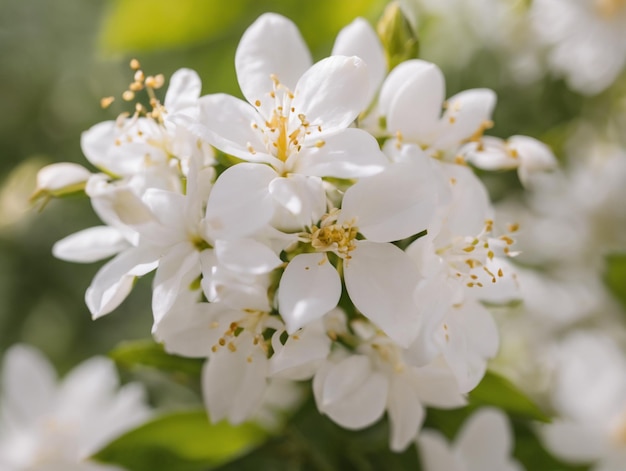This is a detailed close-up photograph of a cluster of beautiful white cherry blossoms. The central focus of the image is on the intricately detailed flowers, which are sharply in focus and clearly showcase their delicate six-petaled structure. Each blossom features vibrant yellow stamens with tiny filaments protruding, dusted with pollen. Surrounding these primary blooms are other buds and blossoms, together forming an impressive cluster of approximately a dozen flowers. The background, slightly blurred, consists of a mixture of greenery and hints of grayish-green hues, enhancing the vibrant foreground. The photograph captures the outdoor natural light of a sunny day, with the clarity of the flowers contrasting against the softer, out-of-focus foliage in the background, highlighting the intricate textures and delicate forms of the blossoms and their oval-shaped leaves. The predominant colors in the image are pure white, soft yellow, and varying shades of green, creating a serene and harmonious composition. The overall effect is a captivating display of nature’s fragile beauty, meticulously detailed in the foreground while becoming more abstract and blurred toward the edges.